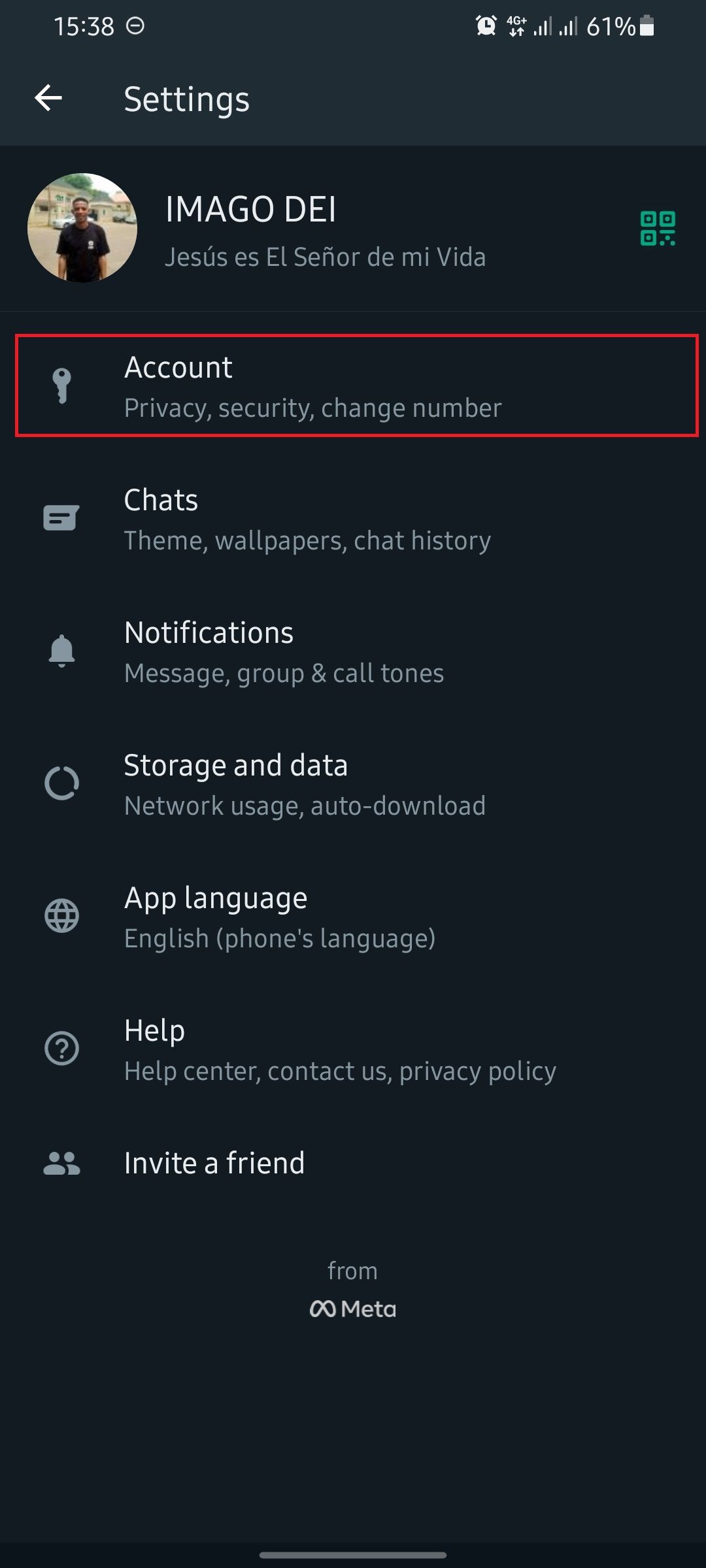The image is a screenshot of a phone taken at 15:38, showing the battery level at 61%. The phone screen is open to the "Settings" section. Prominently displayed at the top is a profile picture of an individual wearing a black shirt and seemingly standing outdoors. Accompanying the image are bold, white letters spelling, "I am a G-O-D-E-I". Below this line, in smaller text and in Spanish, is the phrase "Jesús, El Señor De Mi Vida."

Below the profile details, the "Account" section is highlighted with a red outline, listing various settings options in a vertical format:

- Account
- Privacy
- Security
- Change Number
- Chats
- Theme
- Wallpapers
- Chat History
- Notifications
- Message, Group, and Call Tones
- Storage and Data
- Network Usage
- Auto-Download
- App Language: English
- Help
  - Help Center
  - Contact Us
  - Privacy Policy
- Invite a Friend

At the bottom of the screen, the words "From META" are displayed, signifying the app's association with Meta (formerly Facebook).